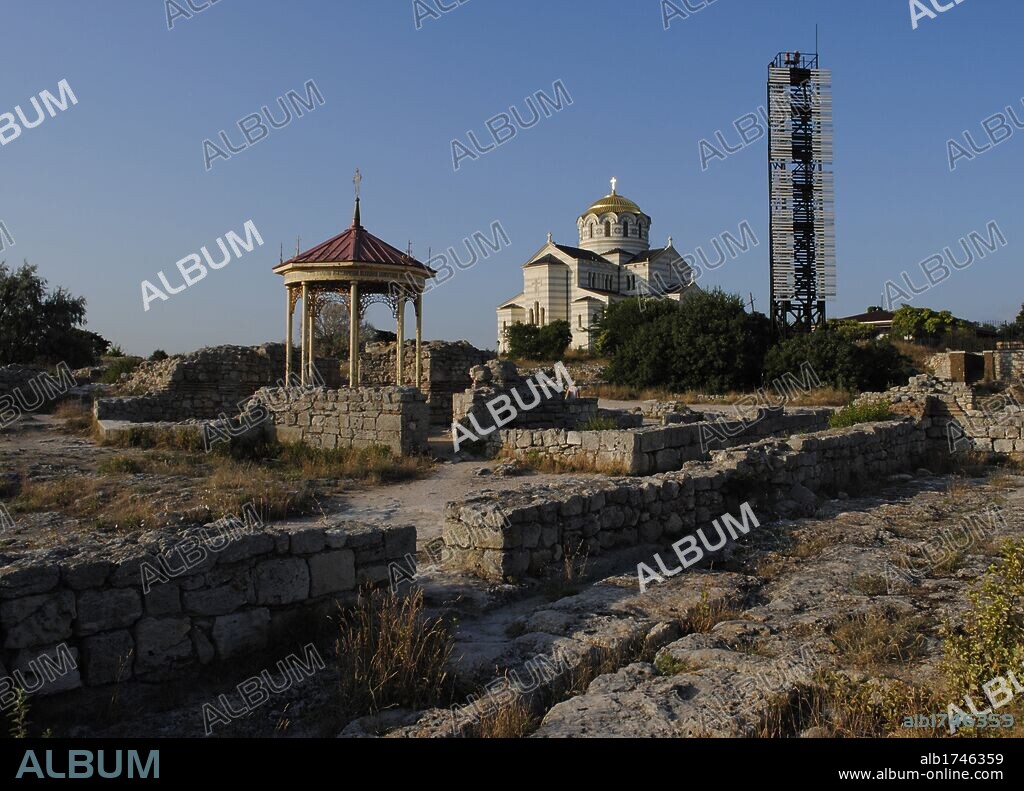The image depicts a professional photograph of a religious structure with a blend of diverse architectural influences. Central to the composition is a large white church in the background, distinguished by a prominent gold dome adorned with a cross, suggesting its significance as a religious landmark. To the left in the foreground stands a gazebo featuring a reddish roof, a cross, and gold embellishments beneath the dome, supported by several columns. The surrounding area consists of various stone walls in different states of disrepair, hinting at an ancient or historical site. Accompanying the scene are patches of greenery, including bushes and trees, along with sparse areas of dead grass and rubble that may have once been part of a garden. A tall, black metal structure resembling a cell phone tower with vertical yellow or silver lines is visible to the right of the church, possibly featuring platforms for maintenance and figures indistinctly perceived atop it. The sky is vividly blue, framing the entire setting. Across the image, the word "album" is watermarked repeatedly in diagonal rows, inscribed in bright white or reverse darker color with a white highlight. At the bottom, there's a black strip displaying "album" in white lettering on the left, with "ALB 1746359" and "www.album-online.com" on the right, also mirrored in teal as a watermark on the image itself.